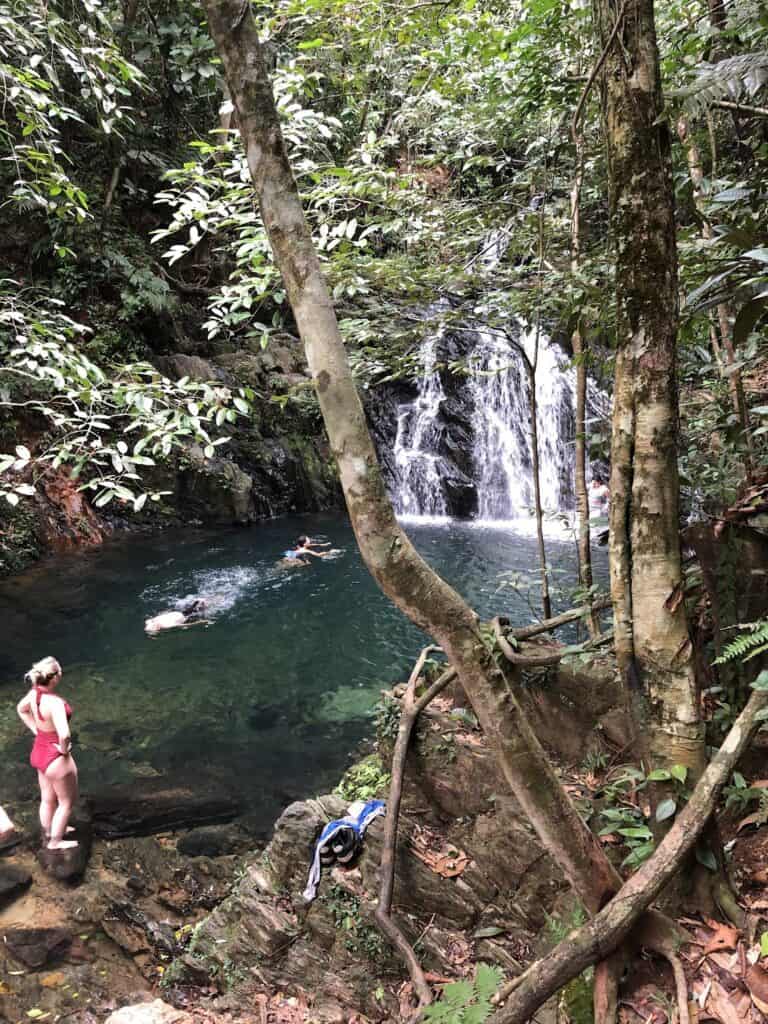In this captivating aerial shot of a tropical jungle, a mesmerizing waterfall cascades down a rocky cliff into a lagoon of crystal-clear blue and green water. The scene is framed by lush vegetation and tall trees with brown trunks adorned with climbing vines and algae. The sunlight filters through, casting a warm glow over the picturesque landscape. Multiple people enjoy the refreshing water; a few are swimming towards the waterfall, while others relax near the shore. On a rocky ledge to the left, a woman with blonde hair, clad in a striking red bikini, stands with her hands on her hips, gazing out at the scenic beauty. Nearby, a pair of black and white shoes and a blue and white towel lie atop the brown rock formation, adding subtle human touches to this serene natural setting.